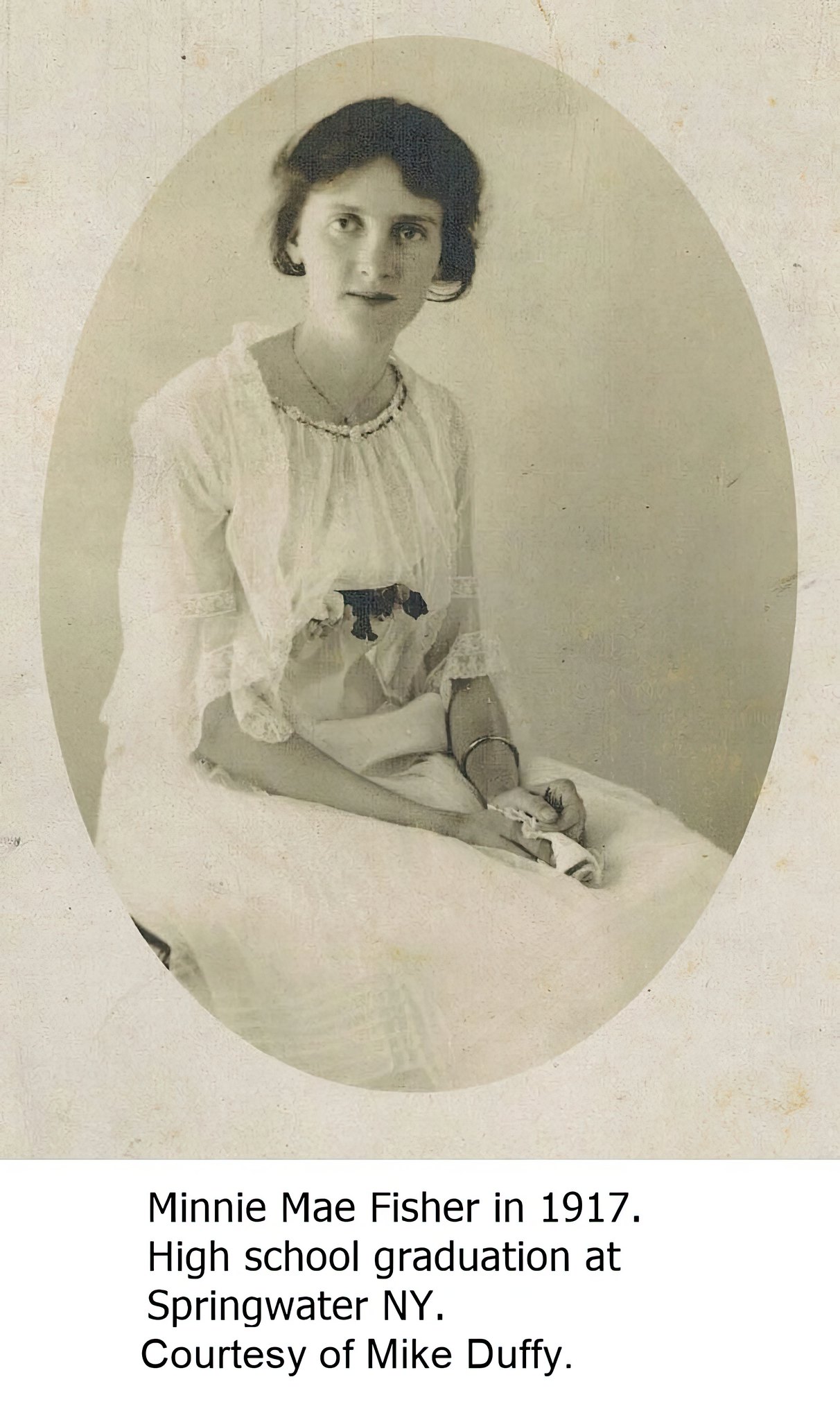This image features an old faded photograph, dated 1917, of Minnie Mae Fisher taken at her high school graduation in Springwater, New York. Provided courtesy of Mike Duffy, the photo is mounted within an oval frame with a beige, stone-like border. Minnie Mae, dressed in an intricate white gown, is seated with her hands gently folded in her lap, holding a white handkerchief. She has short brown hair, likely styled into a bun at the back, and is adorned with a bracelet on her left arm and a necklace. Her serious expression, marked by closed lips, directs a thoughtful gaze forward, while her body is slightly angled to the right. Beneath the image, in black text, the details are inscribed: "Minnie Mae Fisher, 1917, high school graduation at Springwater, New York," highlighting the significance of the moment captured in this historic photograph.